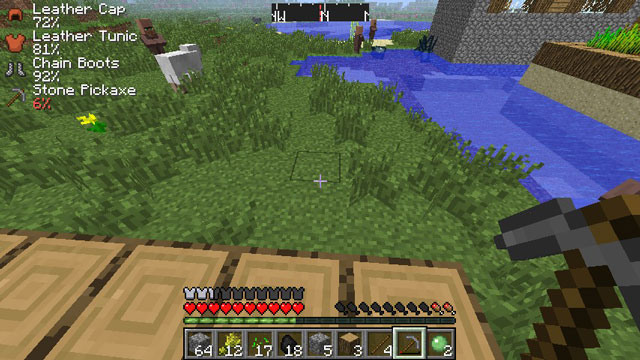A screenshot from a computer game captures a heavily forested area with a moat on the left-hand side, blue water, and structures, including walls and buildings integrated into the water. The upper right section features a building. The center of the screen displays a compass, pointing directly north, within a rectangular interface.

On the upper left-hand corner, there are item indicators: a red icon of a "Leather Cap" at 72%, another red icon of a "Leather Tunic" at 81%, an icon of "Chained Boots" at 92%, and an icon of a "Stone Pickaxe" at 6%. Below these icons and percentages, there's a tan area on the lower left-hand side.

At the bottom, a black bar with a partial green fill appears, followed by red hearts above it. White pieces, some grayed out, are situated above the hearts, indicating various game elements' status. The bottom section also includes a scoreboard displaying: 64, 12, 17, 18, 5, 3, 4, blank, and 2 within individual boxes.